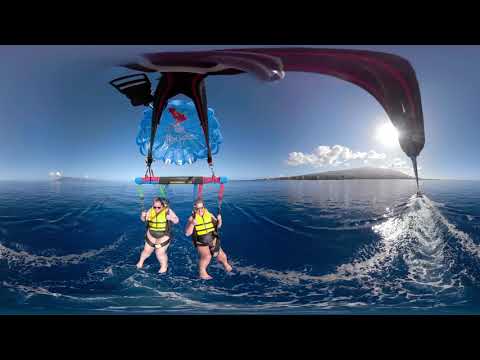This panoramic image captures the exhilarating scene of two people parasailing over a vibrant blue ocean. Both individuals are strapped securely with yellow life jackets and safety belts, hanging beneath a light blue parachute adorned with a red midriff and a black-and-red center lining. The parachute is prominently displayed in the middle of the image, tethered to a boat positioned toward the right side of the frame, which is cutting through the water and creating visible white foam in its wake. To the left and right of the image, distant islands emerge on the horizon, providing a scenic backdrop. The bright sun can be seen partially obscured by a tether connecting the parachute to the boat, illuminating patches of white, puffy clouds that hover over the landmasses. The clean, clear water and the intricate details of the parachute and safety gear are vividly captured, with thick black borders framing the top and bottom of the image.